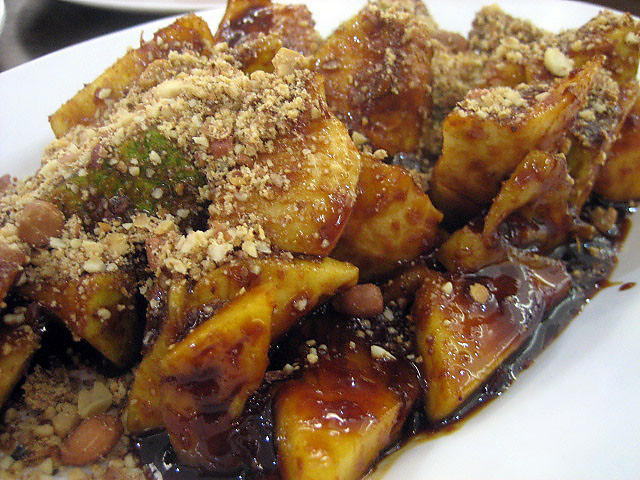This is a horizontal rectangular color photograph featuring a white, undecorated oval plate filled with a dish of food. The dish consists of large, yellowish chunks, possibly fruit or potatoes, coated in a thick, dark brown sauce that appears oily, suggesting the food might be fried. Scattered atop the sauce are light brown crumbles, potentially crumbled nuts or brown sugar, adding texture to the dish. Whole peanuts can be seen embedded within the sauce, particularly noticeable in the bottom left corner. There is also a patch of green underneath some of the crumbles, though it is indistinct. The focus is solely on this plate of food, with no other elements in the background, making it the main subject of the photo.